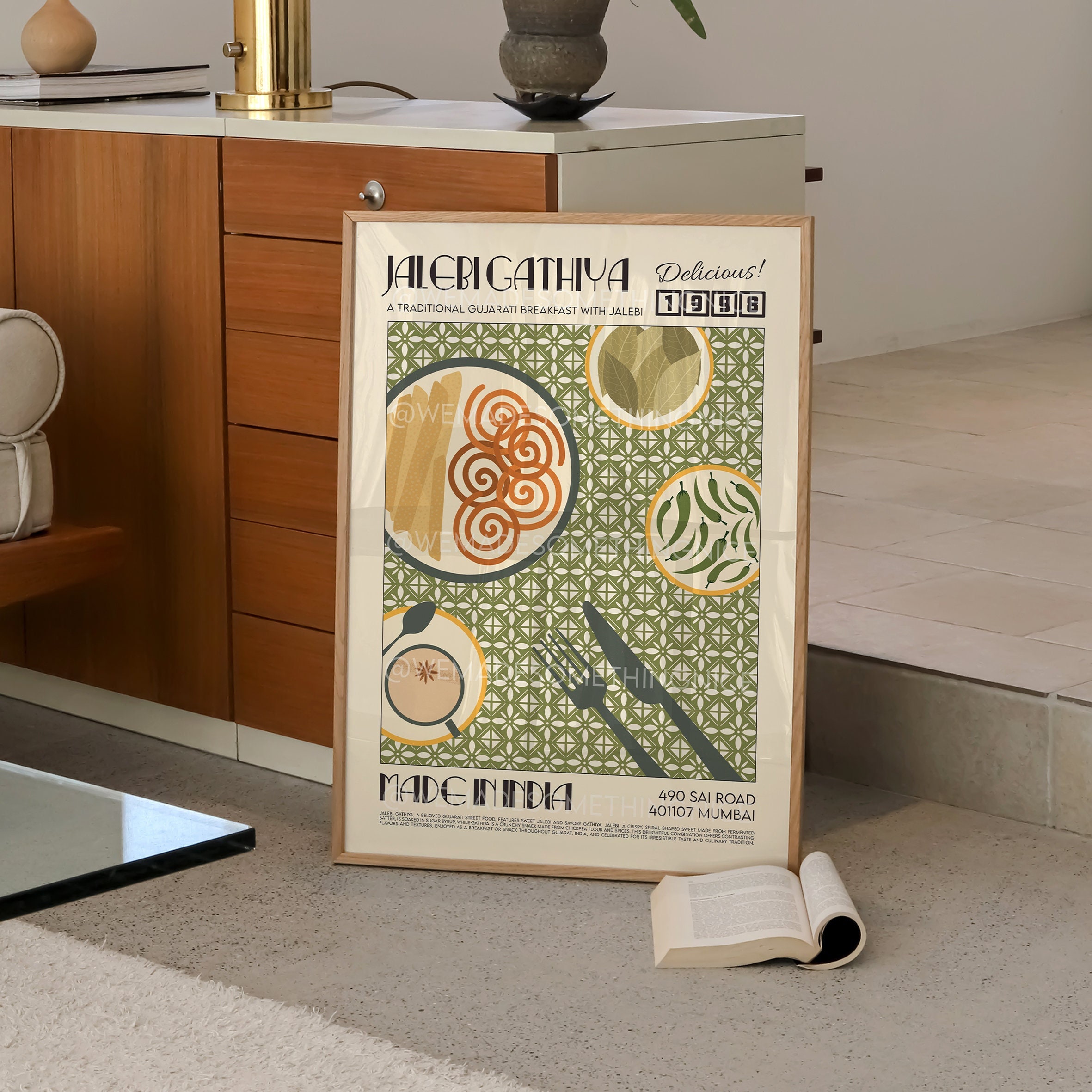The image depicts a staged room setup, resembling a model room from IKEA. Dominating the background is a cabinet featuring a mix of white and dark orange-stained wood with white tops and sides. Directly in front of this cabinet leans a sizeable, colorful poster. The poster advertises a traditional Gujarati breakfast titled "Jalabig Yathia Delicious 1998," showcasing a highly stylized dish with various plates and utensils against a green tiled mosaic background. Additionally, the poster includes the text "Made in India, 490 Sai Road, 401017, Mumbai." In the foreground, there is an open paperback book with its cover tucked underneath. Surrounding the setup are hints of a possible kitchen or living area, including a bit of a glass coffee table and the arm of a couch, all set against muted, somewhat old-fashioned decor.